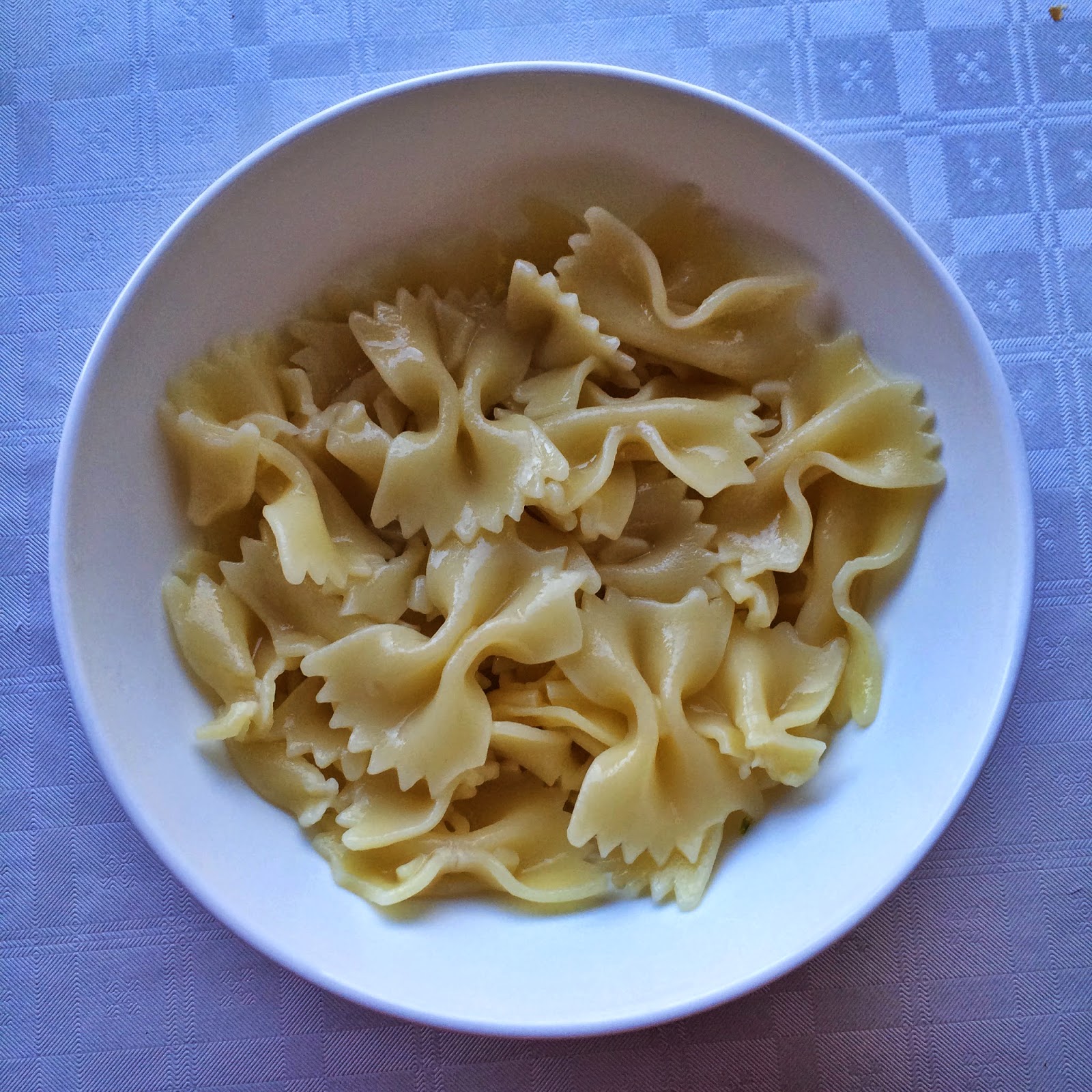This photograph features a white ceramic shallow bowl filled with cooked bowtie pasta, which appears light yellow and slightly glistening. The bird's-eye view emphasizes the perfectly cooked pasta, occupying the entire bowl. The backdrop is a patterned blue tablecloth with various shades of blue, including both squares with little X’s and crisscrossed lines, adding a touch of intricacy. The scene is bathed in natural light, likely from a window, enhancing the appealing texture and color of the pasta. No utensils or additional objects are visible, creating a simple yet elegant presentation of this dish. The image's natural and unedited quality suggests it was taken in a real-life setting, either home or restaurant, during the day.